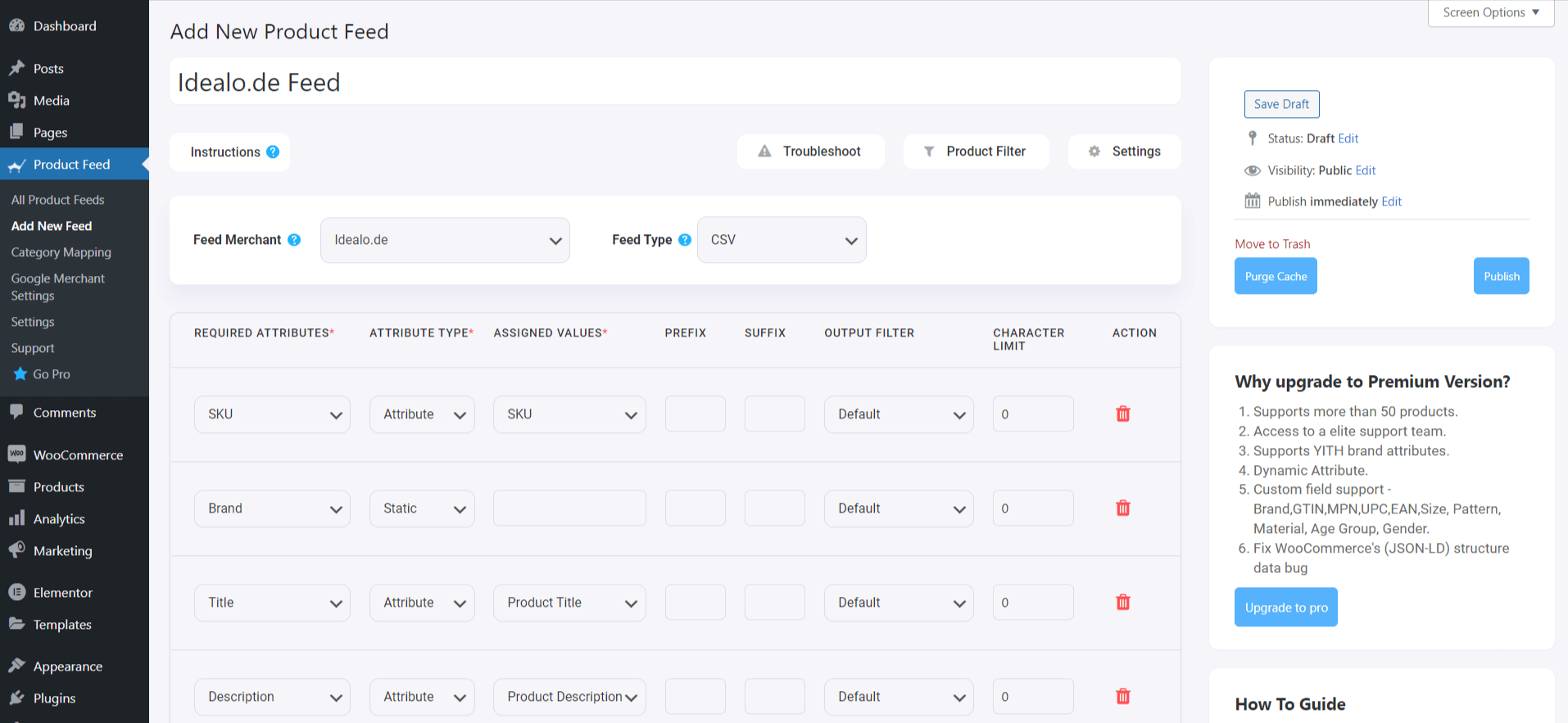The image is a screen capture from a desktop computer, showcasing an application interface. On the left side, a vertical, black-colored sidebar is prominently displayed, featuring an array of options in white text. At the very top of this sidebar is the word "Dashboard." This is followed by options such as "Post," "Media," "Pages," and "Product Feed," with "Product Feed" being distinctly highlighted with a blue bar, indicating it is the current selection. Additional options extend further down the sidebar, though they are not clearly specified.

To the right of this sidebar lies the main section of the application interface, characterized by a clean, white background. The primary heading at the top of this section reads "Add New Product Feed" in black text. Below this heading, the page is organized into several rows, each featuring drop-down boxes designed for user input.

Additionally, on the far right side of the main interface, there are two smaller frames. These frames also have black text and contain blue buttons, indicating interactive elements or primary actions that can be taken within these sections.

The overall layout is intuitive and organized, designed to facilitate the user’s task of adding a new product feed efficiently.